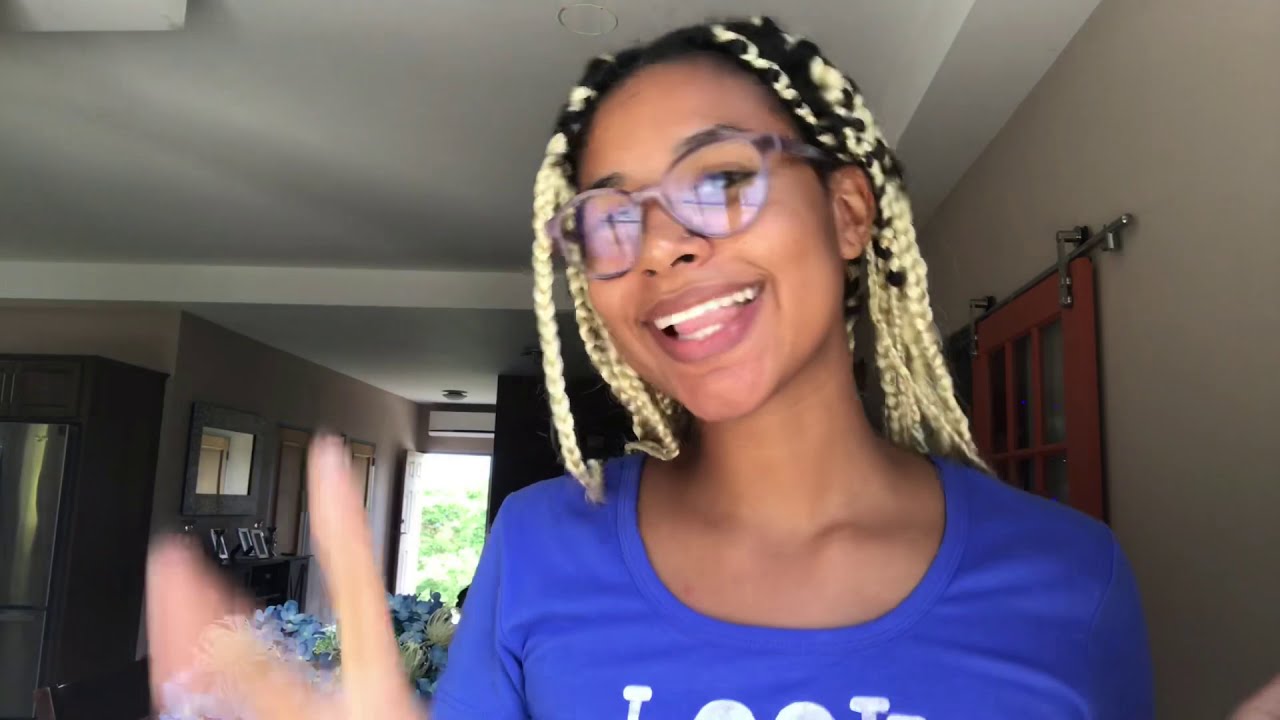The image features a young African-American woman with a radiant, happy smile, her white teeth prominently displayed. She has black hair intertwined with blonde braids, styled into full, neat braids. Her purple-tinted, large round glasses complement her bright purple scoop-neck shirt adorned with partially visible white letters. The woman appears animated, with her right hand blurred, possibly mid-gesture, indicating she's talking energetically. She stands slightly right of center in what seems to be a house. An open doorway with a brown wooden frame behind her reveals green grass outside. To the left in the image, there's a table with purple flowers and green foliage, and further along the wall, there are doors to additional rooms and shelves with picture frames, hinting at a cozy, lived-in space.